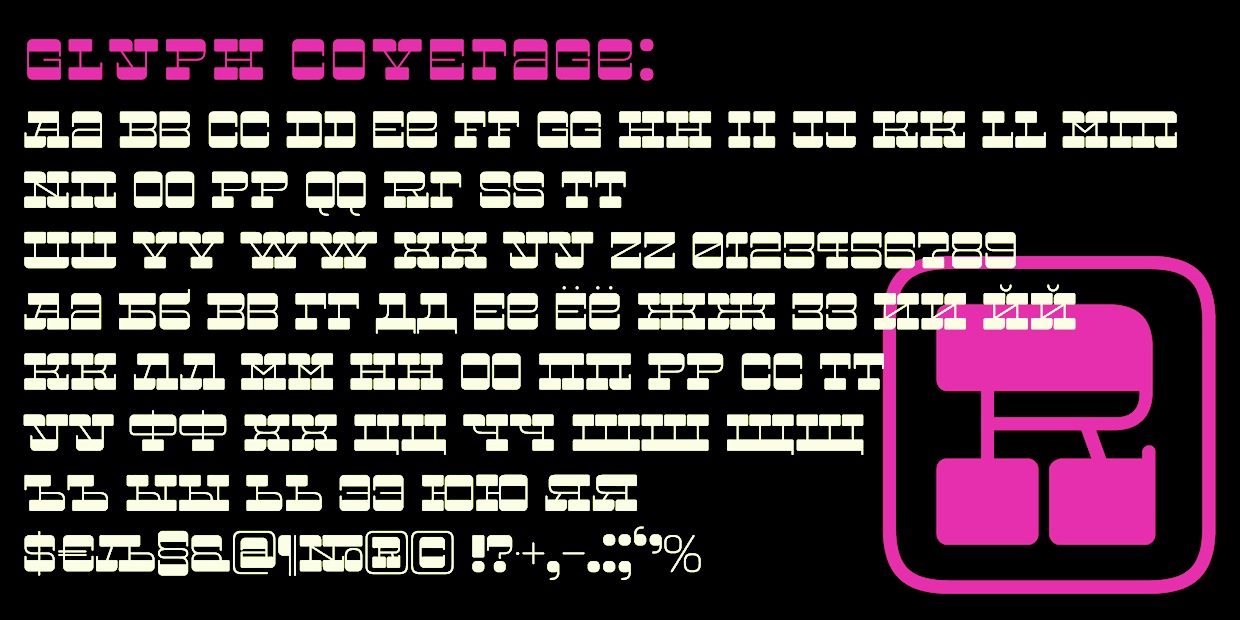This image showcases a surreal and visually striking design. The background is completely black, which contrasts sharply with the vibrant neon pink and white text that dominates the image. At the top, in a unique and unfamiliar font, are the words "GLYPH COYETEEE:" displayed prominently. Towards the lower right-hand corner, an enormous letter "R" in bright neon pink takes center stage, spanning approximately 8 lines in height and about 12 letters in width. Surrounding this central feature is a mix of various letters and symbols from different alphabets, both in capital and lowercase, arranged in 8 lines of white text, creating a chaotic yet intriguing collage.